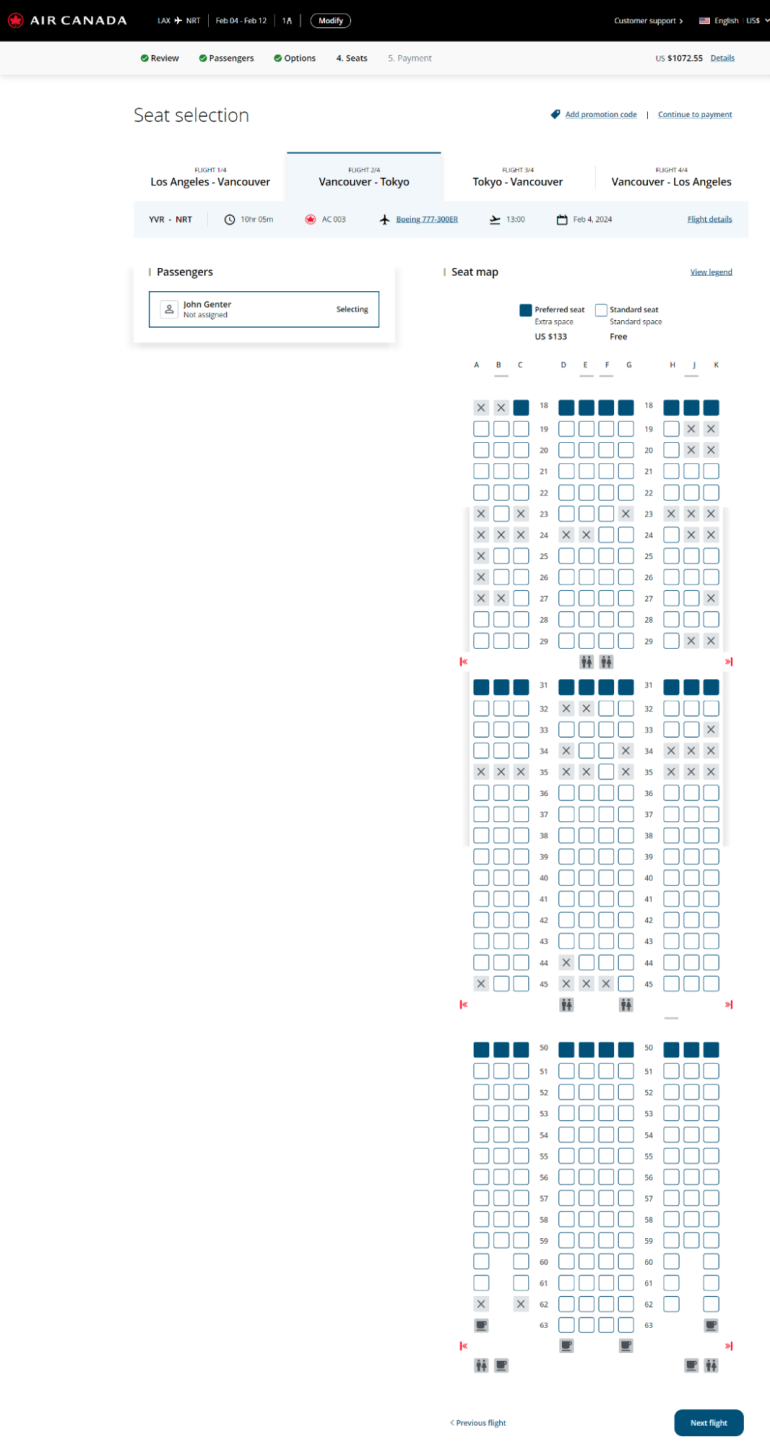The image depicts a screenshot of a cell phone displaying a section of the Air Canada website. At the top, stretching across the entire page, is a black banner with "Air Canada" written in white text, accompanied by the Air Canada logo in the top left corner. A collection of unreadable words are present on either side of the banner, with an English (US) flag and the word "English" next to it in the top right corner.

Below the black banner, the rest of the page features a clean white background. The first horizontal section beneath the banner lists several tabs in white text, which appear to include "Review," "Passengers," "Origins," or "Options," and two other unreadable tabs. To the far right of this section, there are additional unreadable words.

The subsequent line down states "Seat Selection" on the left, with unreadable text to the right. Following this, each leg of a journey is detailed with the respective flight paths: "Los Angeles to Vancouver," "Vancouver to Tokyo," "Tokyo to Vancouver," and "Vancouver to Los Angeles," indicating each segment of a round-trip itinerary.

Further down, although the specifics are unclear, each listed word has a corresponding icon indicating different statuses or options. The following line features two main sections: "Passengers" on the left within a rectangular box with a white background and black writing, presumably listing the names of the passengers. On the right, there is a seat map depicting available and occupied seats from the front to the back of the aircraft.

At the very bottom of the screenshot, there is a blue button with white text that is unreadable, likely intended for a confirmation or continuation action.